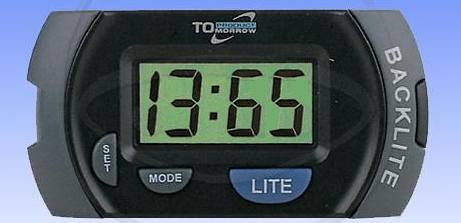This cropped image, likely sourced from product packaging, a magazine, or an advertisement, showcases a portion of a sports style digital watch set against a plain blue background. The focus is on the watch's face, which is bordered in black and partially truncated at the top and bottom edges. On the right side of the watch, there's a small button labeled "Backlight" in white text. The watch face itself features additional buttons labeled "Set," "Mode," and "Light." The digital display, characterized by a green background and black text, prominently shows a time reading of "13.65," resembling a stopwatch format.